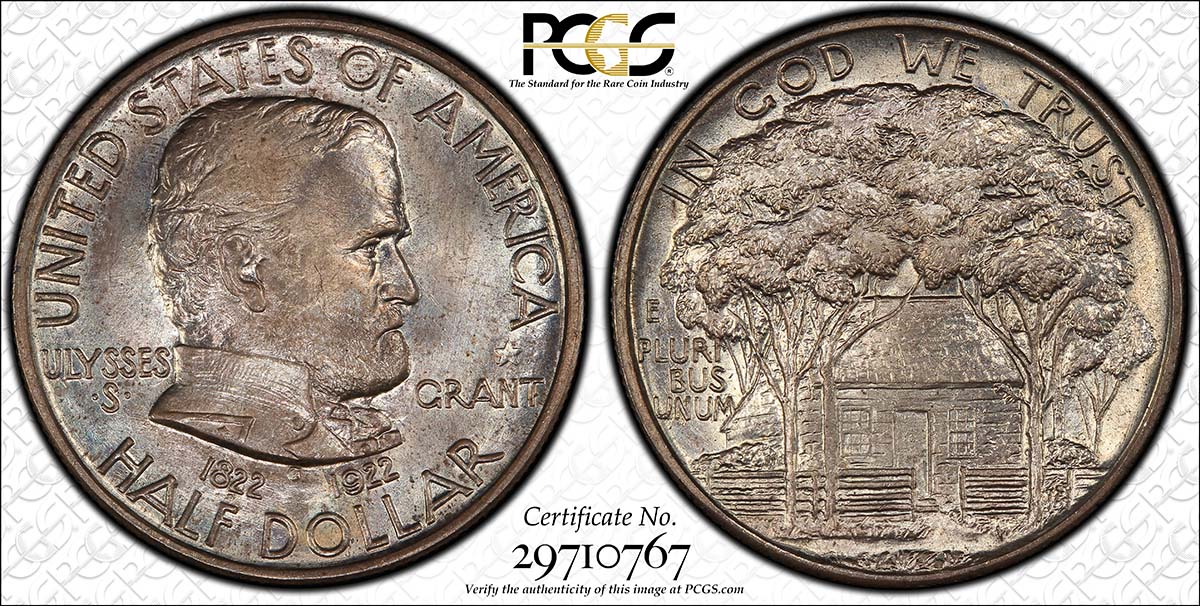This image features a detailed, color photograph in landscape orientation, capturing both the front and back surfaces of a vintage United States half dollar coin, authenticated by PCGS (Professional Coin Grading Service). The main subject is split into two sections: on the left, a side profile of Ulysses S. Grant with his name and the dates "1822-1922" inscribed below. Around the top of the coin are the words "United States of America" and the denomination "Half Dollar" is written across the bottom. The right section shows the reverse side of the coin, depicting a log cabin surrounded by trees, with "In God We Trust" at the top and "E Pluribus Unum" on the left side. In the background lies a rectangular Certificate of Authenticity from PCGS, featuring a repeating logo design diagonally. Centrally placed between the two coin images is the PCGS logo in black and gold, accompanied by the text "The Standard for the Rare Coin Industry." Below, in black text, the certificate number "29710767" is provided along with a prompt to verify the authenticity at PCGS.com. The photograph combines realism with graphic design and typography to present a comprehensive representation of the coin and its certification.